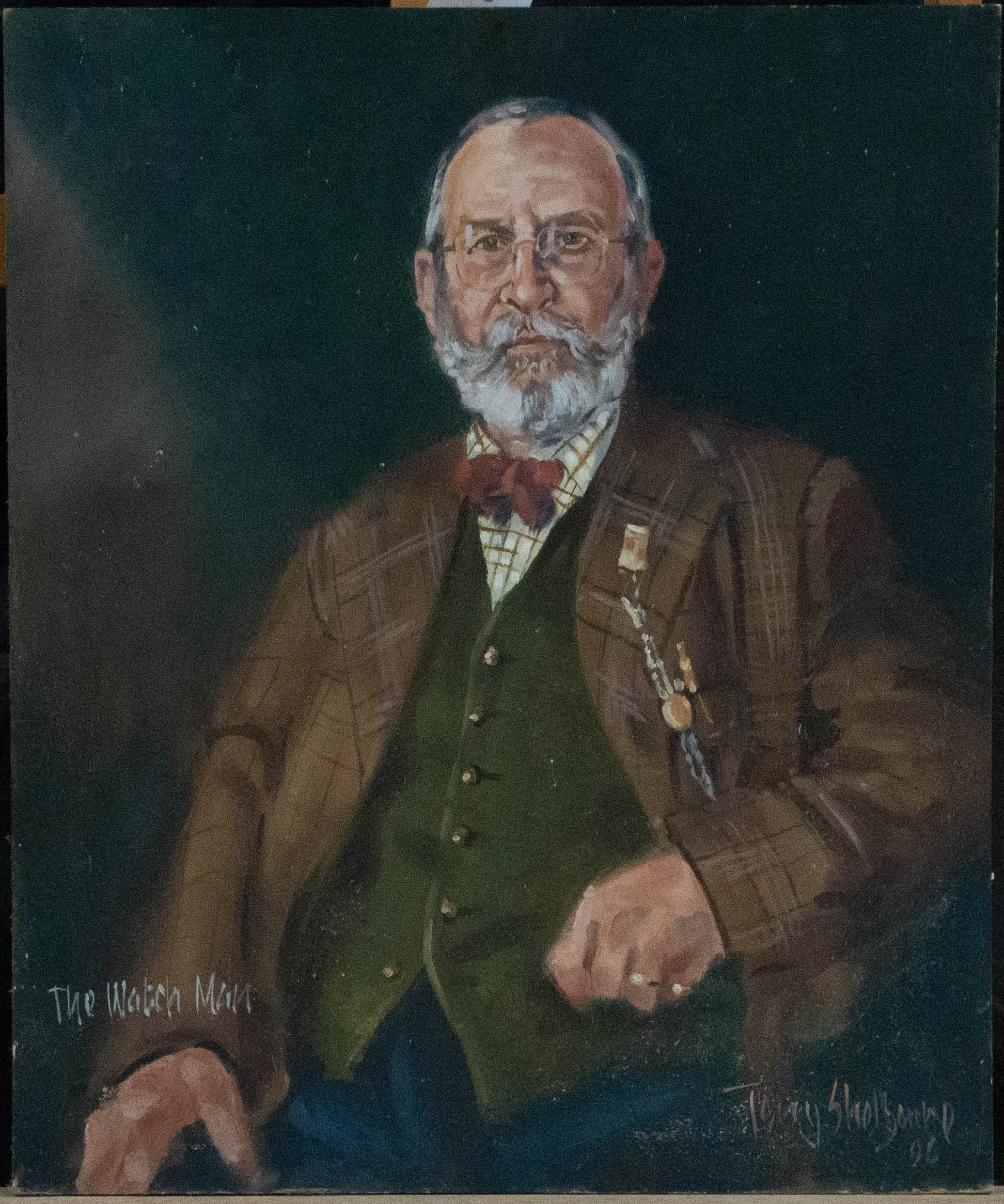The painting, titled "The Watchman," beautifully captures an older gentleman, likely in his 60s or 70s, with a distinctive and detailed appearance. He has a receding hairline and wears large, rimless square glasses that frame his sharp, pointed nose. His facial hair is a striking white beard, tinged with specks of gray, and includes a fluffy mustache that flips out at the ends.

The man is dressed in a meticulously layered outfit, starting with a white and brown striped shirt topped by a red bow tie. Over this, he wears a green vest with a few buttons undone and a checkered brown overcoat with visible chains and ornaments dangling from the pocket. His dark blue waistcoat adds further sophistication to his attire. His hands show a wedding ring and another ring on his pinky finger.

Despite the dapper appearance, his stern expression suggests a reluctance towards having his portrait painted, bordering on irritation or perturbation. The painting is signed at the bottom right, with a notation of '96, while the title "The Watchman" is inscribed on the left.